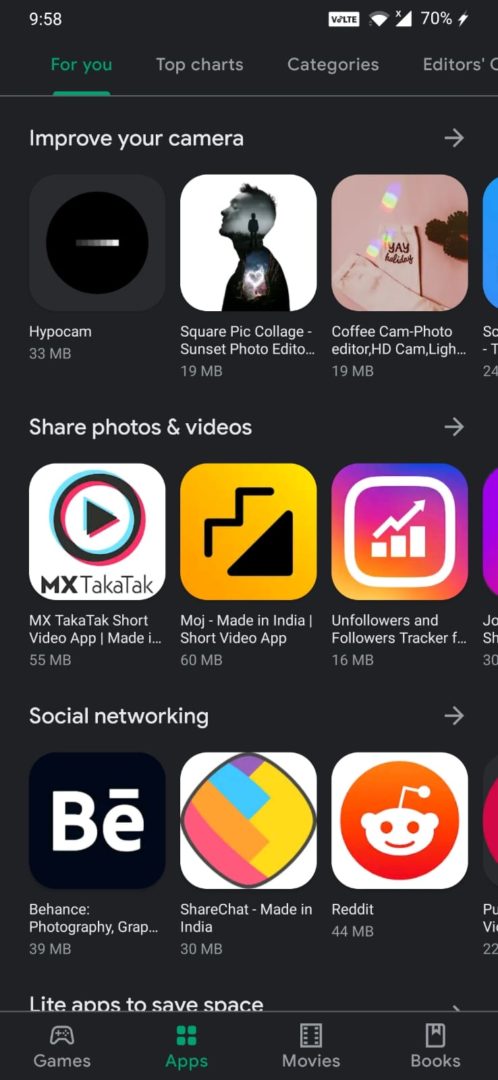The image is a detailed screenshot taken from a music store app interface on a mobile device at 9:58 PM. The phone, connected to WLTE service, has a battery level of 70% and nearly full Wi-Fi signal. At the top of the screen, there are multiple navigation tabs: "4U," "Top Charts," "Categories," and "Editorial Choice," with "4U" currently selected.

In the "4U" section, the display features various app categories starting with "Improve Your Camera," showcasing apps like HypoCam, SquarePic Collage, and Coffee Cam Photo. Following this, there's a category for "Share Photos and Videos," which includes apps such as MX Takataka and Maj Made in India, along with Unfollowers and Followers Tracker. The next category displayed is "Social Networking," listing apps like Behance Photography, Reddit, and Share Chat Made in India.

At the bottom of the interface, different main navigation categories are visible: "Games," "Apps," "Movies," and "Books," with the "Apps" tab currently selected. Additionally, there's a highlighted section titled "Light Apps to Save Space," though no specific apps are visible within this part of the screenshot.